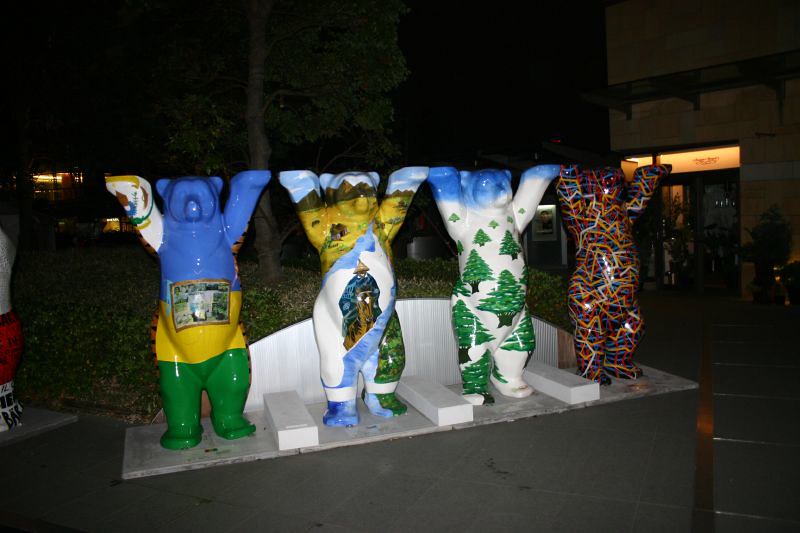This detailed color photograph, taken at night, captures four identically shaped bear figurines, each standing on their hind legs with their front paws raised as if to support a flat object above them, such as a plate. The backdrop is a stark black sky, contrasting with the illuminated figures and hinting at an urban setting with faintly visible buildings and street elements in the background. One building is on the upper left with indistinct features and lights, while another, possibly a storefront, is on the upper right with under-awning lighting. The bears stand on a large gray structure interspersed with white rectangular prism blocks separating each figure.

From left to right, the first bear is painted in a gradient of blue at the top, transitioning to yellow in the middle, and finishing with green at the bottom. The second bear features an abstract desert mountain scene with blue and white sky and earth tones for the mountains and trees. The third bear depicts a snowy landscape adorned with distinct Christmas trees, painted in white and green. The fourth and final bear is covered in dark brown paint accented with vibrant multicolored angular squiggles, giving it a striking appearance. The overall setting includes a grassy median and hints of the asphalt road below, adding to the night-time urban ambiance.